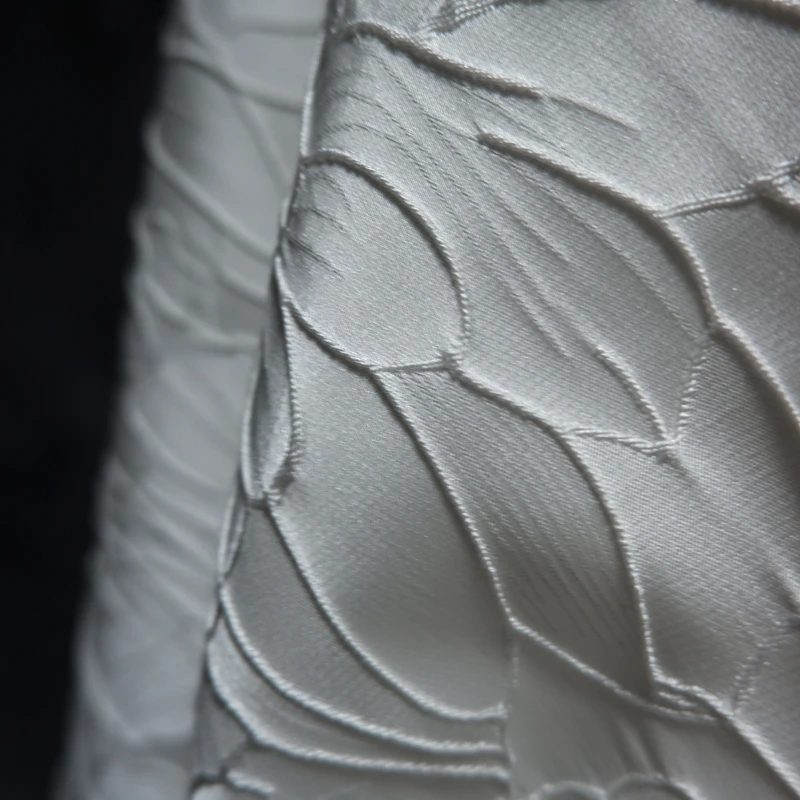A detailed image features a white cloth adorned with intricate leaf designs. Each leaf is meticulously bordered with white, enhancing its shape against the backdrop. The cloth's background is a deep black, which appears slightly blurry, adding a sense of depth to the image. The fabric has a subtle shine, contributing to its elegant appearance. Additionally, fine white threading interlaces across the surface, adding another layer of texture and complexity to the overall design.